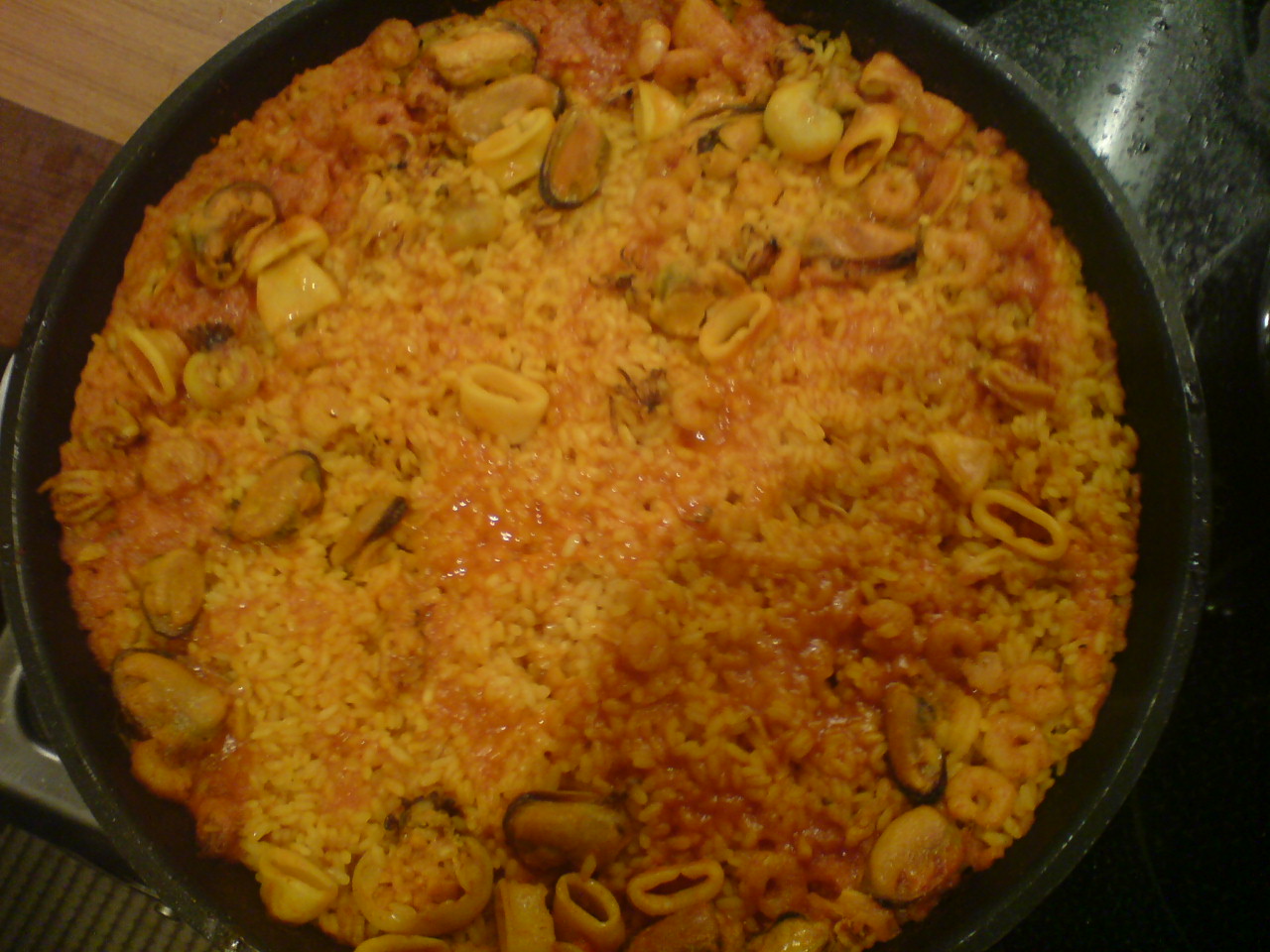This photograph captures a detailed overhead view of a culinary dish being cooked in a black cast iron pan, which is placed on a wooden countertop or possibly a stove. The dish appears to be a vibrant yellowish-orange paella, featuring a mix of rice, circular pasta, vegetables, potential jalapenos, shrimp, and other seafood that could include mussels or oysters. The pan occupies most of the image, with wood visible in the top left corner, suggesting it rests on a counter. In the top right, there seems to be either a handle or a part of a stove, both of which are black. The bottom left edge of the image reveals part of a metal buckle, possibly related to the end of the stove, and below that, part of what appears to be the edge of a floor mat or rug presents itself, characterized by dark coloring. The bottom right corner remains pitch black, providing no additional details. Overall, the scene vividly showcases the preparation of a hearty paella in a kitchen setting.